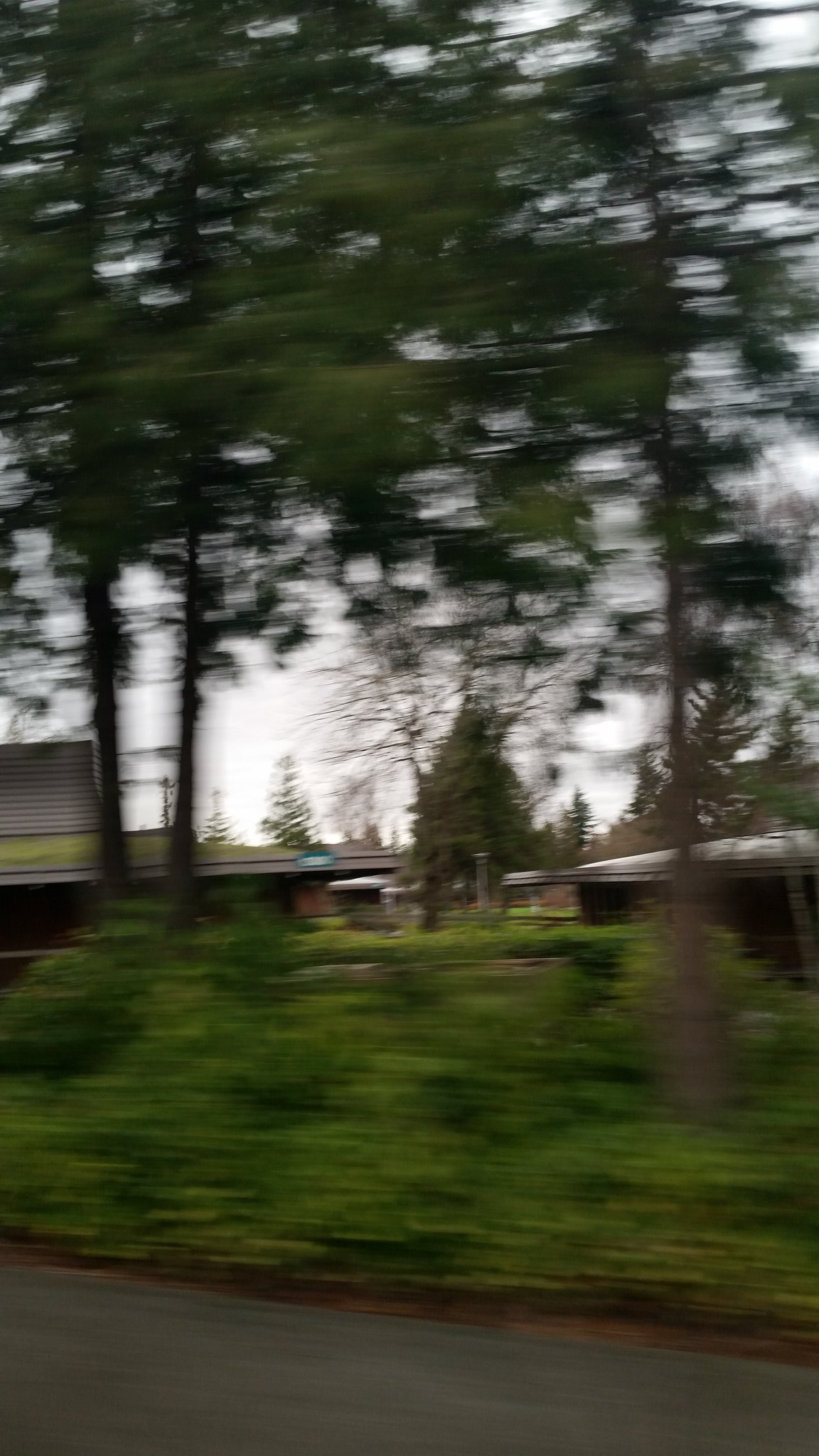The image is a blurry photograph taken from a moving car, capturing an outdoor scene with noticeable motion blur. In the foreground, there's a light black or grayish roadway bordered by some green grass and shrubs. Tall pine trees with green leaves can be seen on both sides and in the background of the image. In the distance, low, long, one-story buildings with roofs of varying colors, such as white and green, reminiscent of a strip mall or stores, are visible. Overall, the scene is predominantly green and characterized by the natural elements of trees and bushes along with the man-made structures in the background.